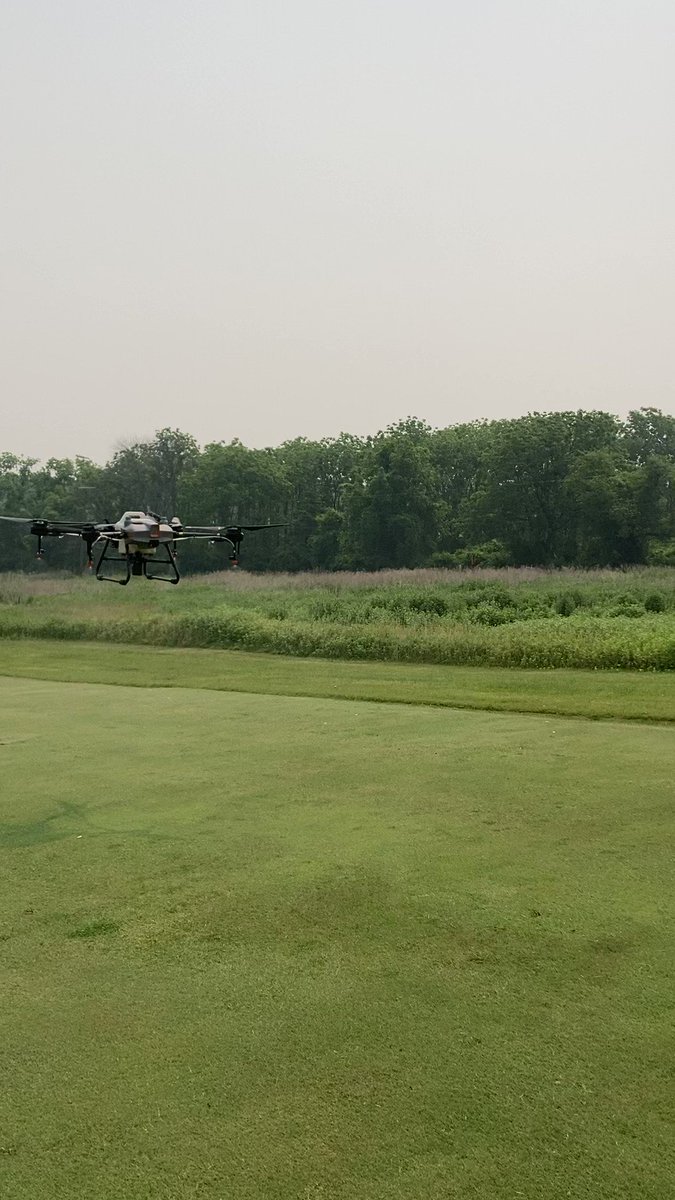The image depicts a large vertical photo capturing a drone in mid-flight over a meticulously maintained landscape that resembles a golf course. In the foreground at the bottom of the photo, there is closely cropped green grass, transitioning into a slightly taller semi-rough area that spans about two feet, and further into shin-high rough grass. This leads into the mid-background dominated by a dense line of trees stretching across the upper middle section of the photograph. The sky above is a uniform gray with no visible individual clouds. The drone, situated on the center-left side of the image, has a white body with black slats underneath and black rotors, along with two brackets and a front-facing camera. The drone's precise positioning and details are clearly visible, flying close to the ground without any textual or human/animal presence in the photo.